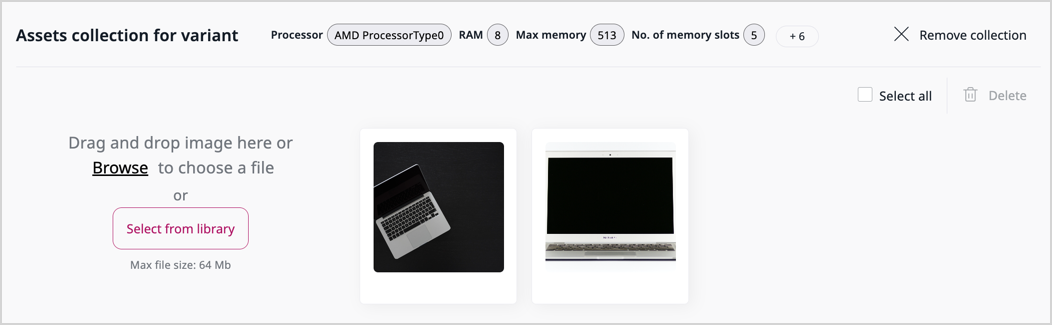This image features a user interface for managing image collections. It showcases two distinct sections, each represented by a gray, rectangular box.

### Top Section: 
1. **Collection Label**: Each gray box is labeled "Collection" in the top corner.
2. **First Image Collection**: Titled "White," this collection includes:
   - **Instruction Text**: "Drag and drop image here or browse to choose a file or select from library."
   - **File Size Indication**: The size of the files is displayed.
   - **First Image Description**: A clean, modern home office featuring a white desk.
   - **Second Image Description**: Another home office setup with two monitors on a white desk.
3. **Top Section Options**: 
   - **Remove Collection**: An option to delete this collection.
   - **Select All**: A button to select all images in this collection.
   - **Delete**: A circular button for deletion.

### Bottom Section:
1. **Collection Label**: This section is also labeled "Collection."
2. **Second Image Collection**: Titled "Oak and Black," this collection includes:
   - **Instruction Text**: "Drag and drop image here or browse to choose a file or select from library."
   - **File Size Indication**: The size of the files is displayed.
   - **First Image Description**: A brown desk situated in an office with a wooden floor. The window view includes leafy trees.
   - **Second Image Description**: Another brown desk in front of white walls, featuring a monitor with accessories, a dark-colored chair, and a brown floor.
3. **Bottom Section Options**:
   - **Remove Collection**: Located in the upper-right corner with an 'X' icon for deletion.
   - **Select All**: A button to select all images in this collection.
   - **Delete**: A circular button for deletion.

This detailed interface preview provides an organized and visually coherent way to manage and view office setup images, with intuitive options for removing and selecting images.